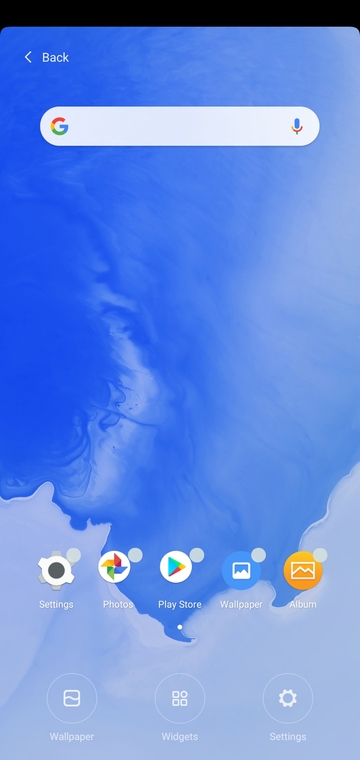The image depicts a minimalistic Android wallpaper that presents an intriguing visual ambiguity. At first glance, it appears to be a view of the sky, but on closer inspection, it resembles an aerial perspective of a vivid blue body of water surrounded by ice, akin to a frozen lake. The scene is predominantly blue, with the ice creating a defined boundary around the water.

Overlaying this wallpaper are five icons: Settings, Photos, Play Store, Wallpaper, and Album. Each icon features a small gray badge, possibly indicating recent updates. Positioned at the top left is a back button, whose presence suggests an ongoing navigation session. At the bottom of the screen, transparent buttons labeled Wallpaper, Widgets, and Settings suggest an active overlay that can be customized. Additionally, the Google search bar, capable of voice input, is placed at the top.

The middle section of the screen is notably sparse, emphasizing the minimalist design of the wallpaper. The overall layout blends functionality with a visually intriguing background, creating a unique and interactive user interface.